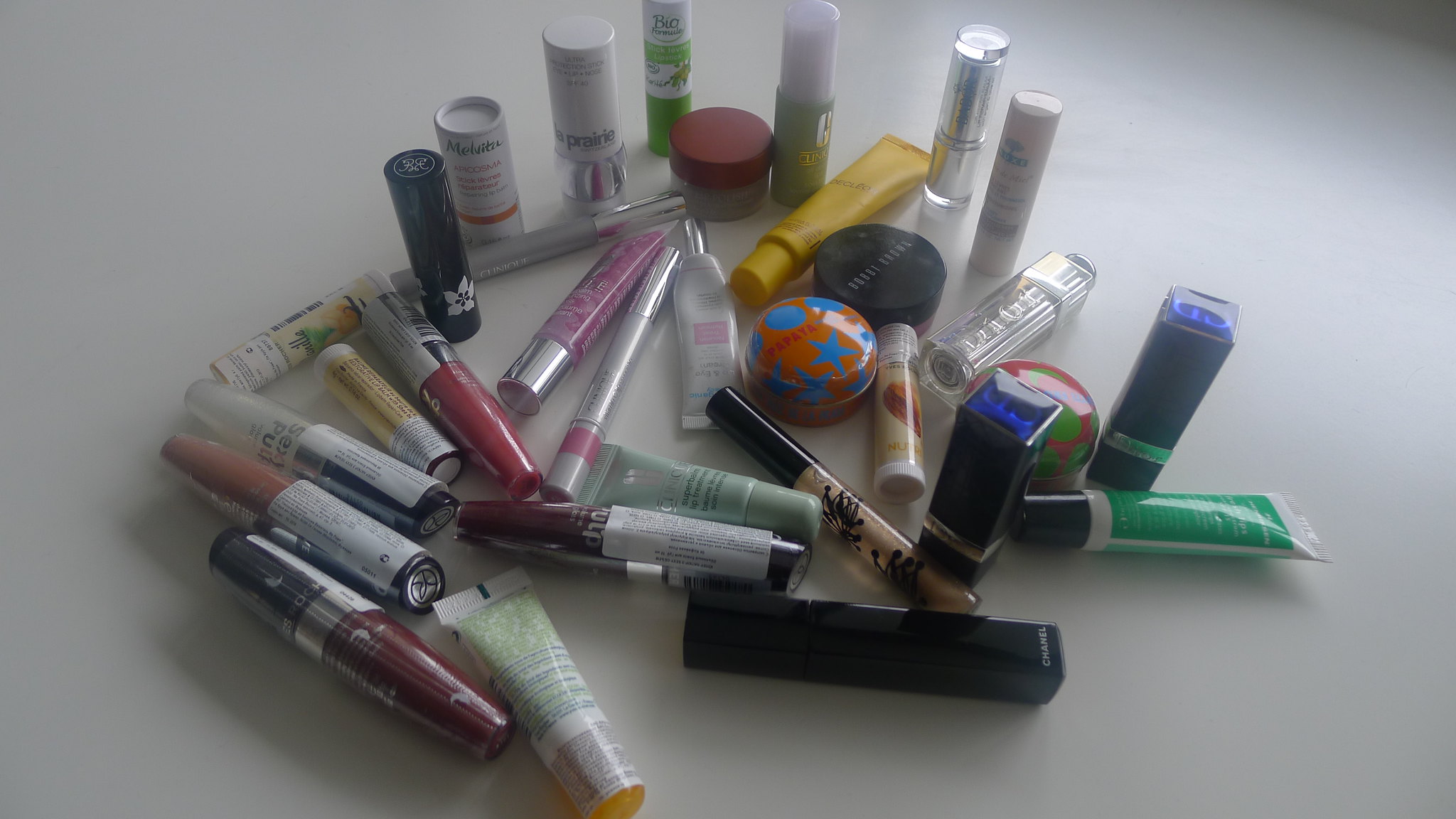This photograph showcases an array of makeup and cosmetic products meticulously arranged against a pristine white background. The lighting is brighter towards the rear of the image, casting soft shadows that extend towards the lower left corner. The composition features a diverse assortment of items, including several lip products predominantly located at the bottom left, lying elegantly on their sides. The majority of the products are positioned upright, flaunting a variety of colors, designs, and styles.

Among the collection are sleek, long thin tubes alongside thicker cylindrical containers, indicative of different cosmetics like lipsticks, chapsticks, and lip balms. Some products have a circular shape, while others boast a more boxy appearance. Notably, a few items display recognizable branding, with identifiable Clinique’s distinct coloring and logo, and a classic Chanel piece standing out amidst the colorful array. This detailed assembly illustrates a vibrant and eclectic mix of contemporary cosmetic essentials.